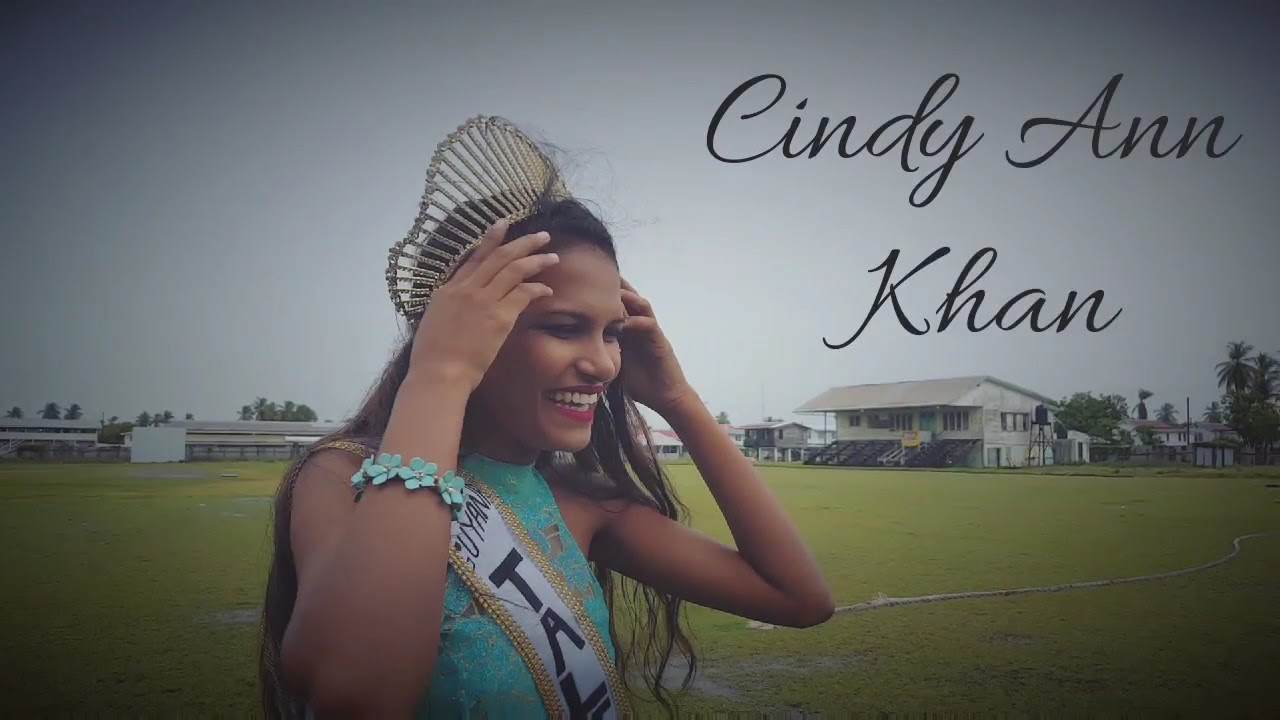The image depicts a tanned-complexioned woman wearing a gold, roller coaster-shaped crown and a sleeveless, bluish-greenish, or teal dress. She has long black hair and is smiling or laughing, creating a joyful demeanor. Across her torso, she wears a sash reminiscent of a Miss America pageant, emblazoned with "GUYAN" in black letters. On her wrist, she sports a bracelet featuring turquoise flowers. She stands slightly to the left, facing right and somewhat forward, against a backdrop of a big grassy field dotted with houses and scattered palm trees.

In the distance, to the left side of the image, several small buildings can be seen. On the right side, there is a prominent two-story building, possibly with bleachers in front. Additionally, a few trees appear in the background on the right. The sky above is gray and stretches across the upper portion of the image. Written in black cursive in the upper right corner is the name "Cindy Ann Khan," positioned against this sky.

The scene is bathed in natural daylight, suggesting that the photo was taken during the daytime.